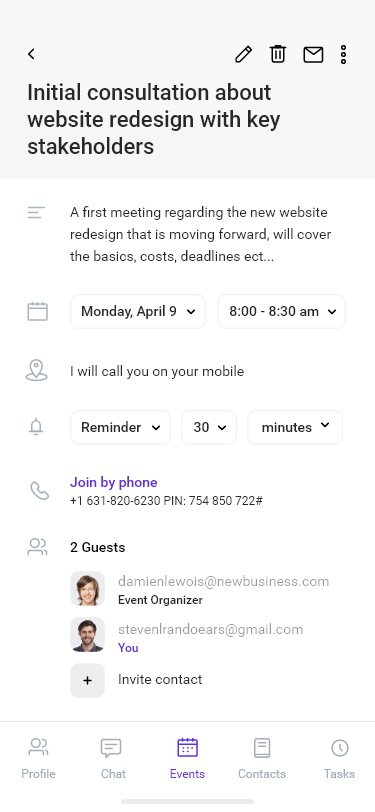### Detailed Screenshot Description

The screenshot captures an event page detailing an initial consultation meeting about a website redesign with key stakeholders. At the top-right corner, there are three icons: a pencil, a trash can, a mail icon, and a set of three dots indicating additional settings.

### Header
- **Title**: "Initial Consultation About Website Redesign with Key Stakeholders"
  - Displayed in large, bold black text.

### Description
- **Summary**: 
  - A brief paragraph in dark gray text states: "A first meeting regarding the new website redesign that is moving forward will cover the basics, costs, deadlines, etc."

### Event Details
- **Date and Time**:
  - Displayed with a calendar icon: "Monday, April 9th, 8:00 AM to 8:30 AM."
  
- **Location**:
  - Indicated by a location pin icon: "I will call you on your mobile."

### Alerts and Access 
- **Reminder**:
  - An alert icon with text: "Reminder, 30 minutes before."
  
- **Phone Access**:
  - A phone icon with blue text: "Join by phone" followed by the black text phone number.

### Attendees
- **Guests**:
  - Depicted by a people icon indicating "2 guests."
  - Icons and names:
    - Damian Luis (email: damian.luis@newbusiness.com)
    - Steven L. Ren Doears (email: steven.ren@gmail.com)

### Footer Icons
- At the bottom of the screen, several icons are displayed:
  - **Profile icon**
  - **Chat icon**
  - **Events icon**
  - **Contacts icon**
  - **Task icon**

This detailed layout covers all essential information about the meeting, providing a clear and organized view of the event's specifics.